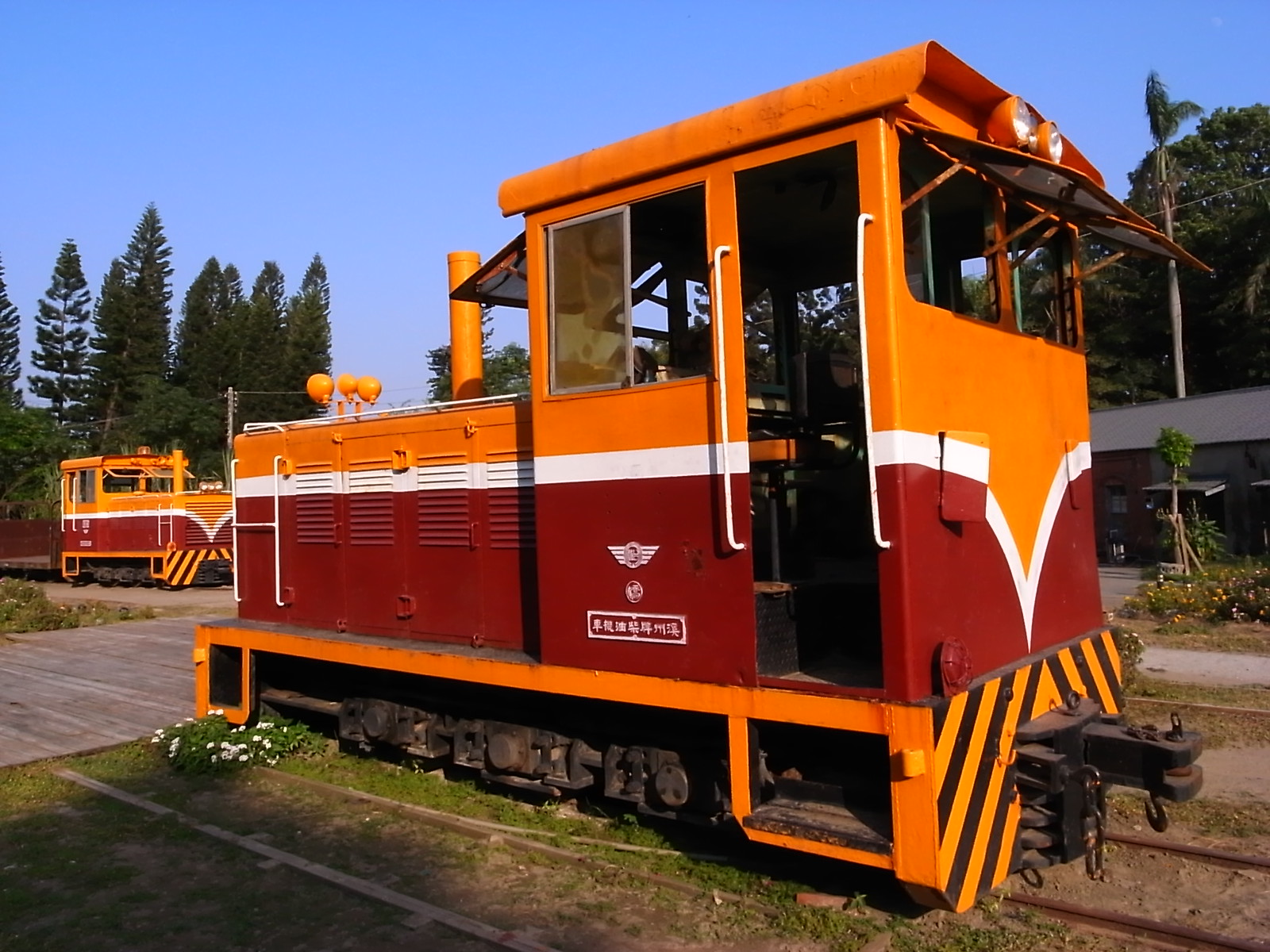The image depicts an old, decommissioned train engine with a predominately orange body, accented by a reddish bottom and separated by a white strip that narrows to a point at the front. The engine, with open windows and doorframes, includes compartments for the conductor. It rests on train tracks surrounded by patches of dirt and grass. A wooden walkway is visible behind it. In the background, an identical train car faces the opposite direction on a separate track. Surrounding the scene are a building to the right, trees along the horizon, and a clear, cloudless blue sky, suggesting a sunny day.